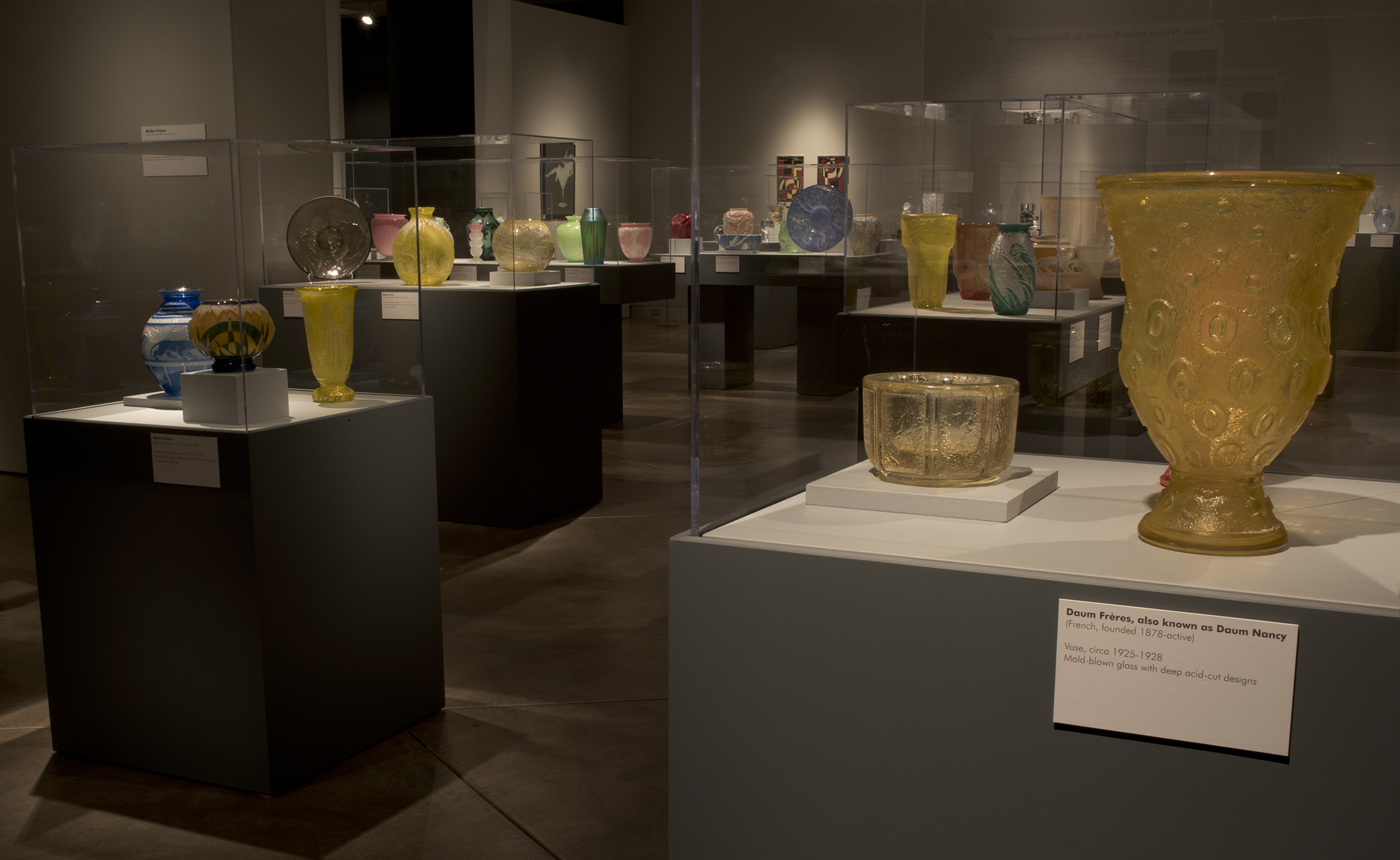The image captures the inside of a dimly lit museum or art gallery specializing in glassware or ceramics displays. The gallery features gray walls and a dark brown floor. The exhibits are illuminated by overhead lights, providing contrast and focus to each piece. Scattered throughout the room are large, square-shaped, gray pedestals with white tops, some encased in glass covers. 

Prominently seen on the left side of the image, one pedestal displays three vases: one blue and white, one gray and black, and one yellow. On the right side, the closest pedestal to the camera showcases two vases—a small, semi-clear gold-colored vase, and a larger yellow vase. The smaller vase has intricate acid-cut designs attributed to the Dume Frères, also known as Dume Nancy, renowned French artisans active from 1878 to 1928. This specific piece, mold-blown glass with deep acid-cut designs, dates back to approximately 1925-1928. A white card with black writing is affixed to the front of the pedestal, providing details about the pieces.

In the background, more vases in various colors, including yellow, blue, green, pink, and magenta, are displayed on similar pedestals, also enclosed in glass cases. Several framed pictures hang on the walls, adding to the aesthetic and historical ambiance of the setting.